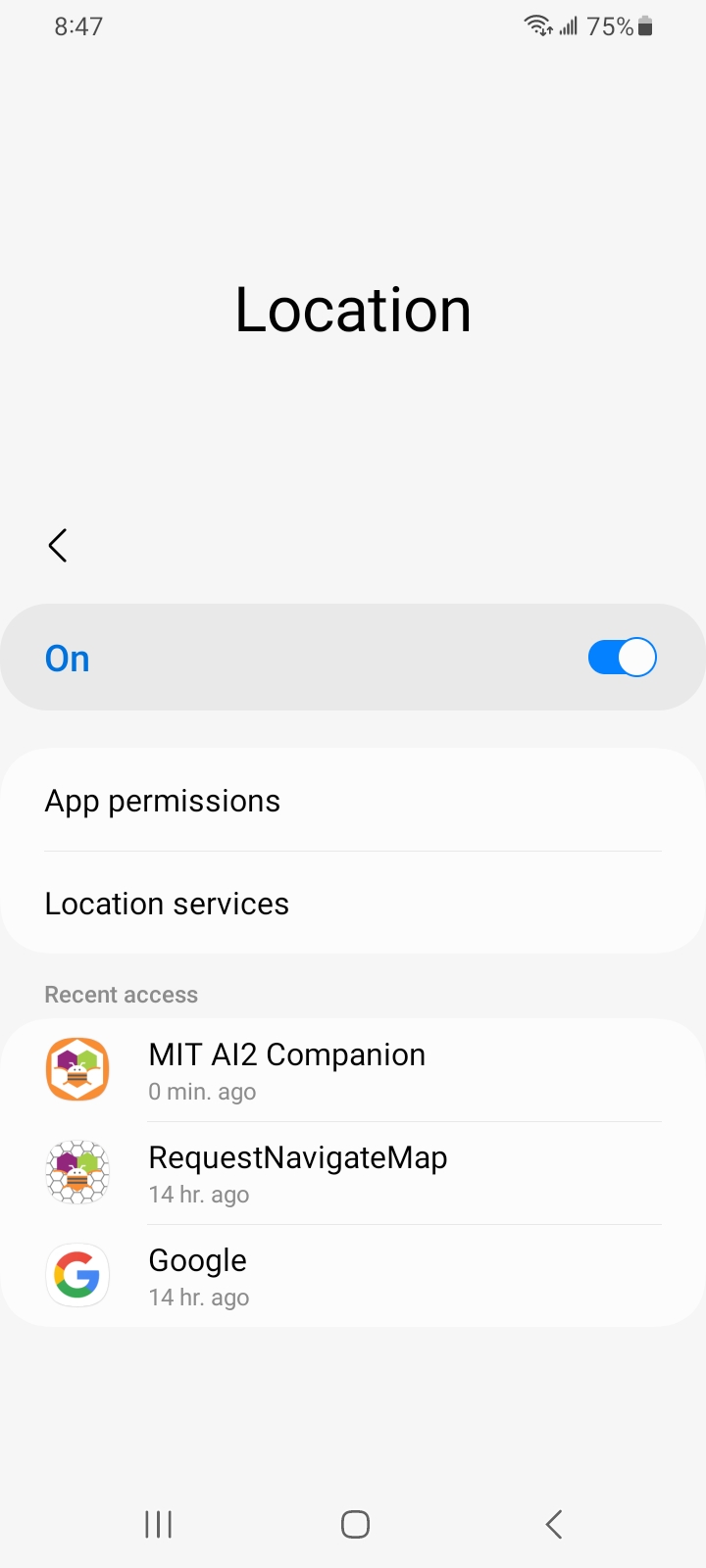The image showcases a detailed interface layout of a light-gray rectangular screen. 

At the top-left corner of the screen, there's a digital clock displaying "8:47". On the top-right corner, a signal strength icon is visible with progressively taller bars towards the right, indicating Wi-Fi connectivity. Adjacent to this, the battery icon shows 75% charge remaining.

In the center of the screen, the word "Location" is prominently displayed. Below this, on the left-hand side, there is an arrow pointing to the left, accompanied by a darker gray bar labeled "On," which is highlighted in blue. To the right of this bar is another blue bar with a white circle outlined in blue, adjacent to the text "App Permissions, Location Services, Recent Access."

Moving further down, there is an orange symbol with intersecting brown, green, and purple segments labeled "MIT A12 Companion, 0 MIN ago." Below this is another symbol composed of small white circles and variously colored shapes (purple, green, and orange), annotated with "Request Navigate Map, 14 HR ago." Following that, the familiar multicolored Google "G" logo appears, with the text "Google, 14 HR ago" beside it.

At the bottom of the screen, another gray rectangular section is present. On the left-hand side of this section, three evenly spaced horizontal bars are depicted, next to a square with rounded corners and an arrow pointing to the left inside it.